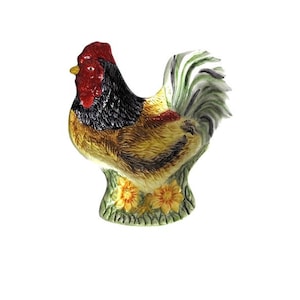The image depicts a small ceramic rooster statuette set against a plain white background. The rooster is facing left, displaying its full left side. Its head, comb, and eyes are a dark cherry red, with a small yellow beak. The neck is dark brown, while the body is predominantly light tan with some darker feathering. The tail is bushy, featuring a mix of white, light green, and black feathers. The base of the figurine mimics grass, painted green and adorned with two yellow daisy-like flowers, each with burnt orange rims. The statuette’s intricate detailing, from the textured body to the colorful and elaborate feathers, captures the essence of a proud and vibrant rooster.